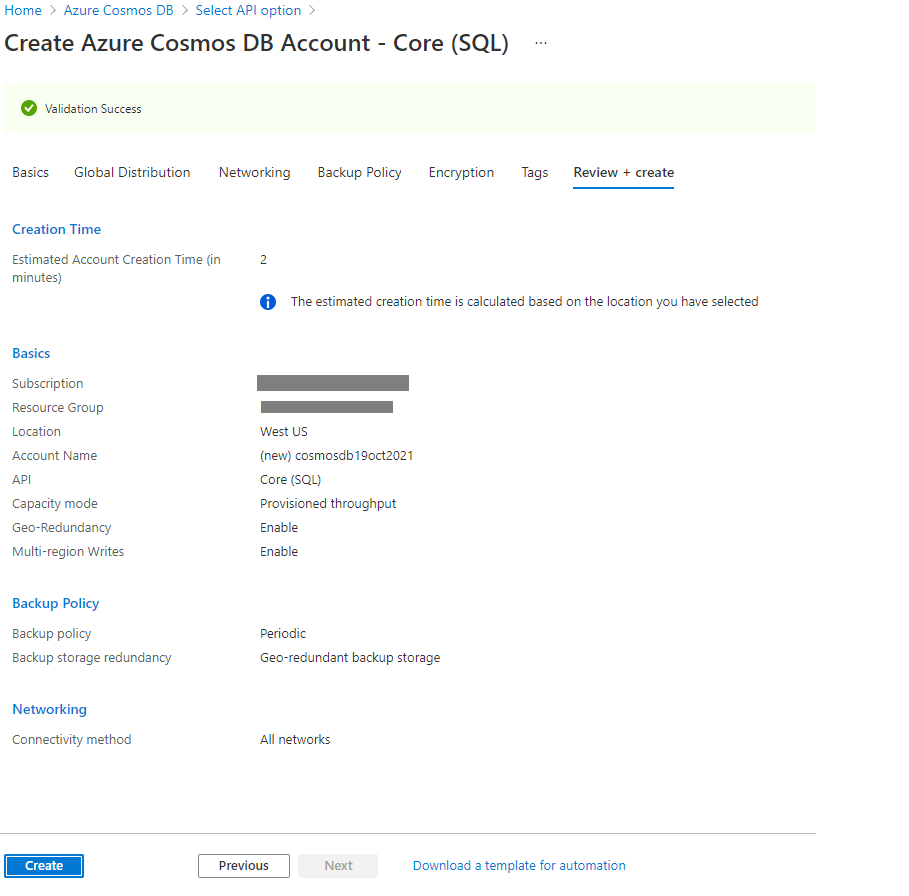The image displays a user interface for creating an Azure Cosmos DB account. At the top, are the headings in blue text: "Home", "Azure Cosmos DB". The user has selected the "API" option, indicated by the text "Create Azure Cosmos DB Account - Core (SQL)".

A green circle with a checkmark denotes "Validated Success". Beneath it, tabs are labeled: "Basics", "Global Distribution", "Networking", "Backup Policy", "Encryption", "Tags", "Review + Create". The "Creation Time" section follows, with "Estimated Account Creation Time" and a clickable input for entering the estimated time based on the selected location.

The "Basics" section includes fields for "Description", a grade bar for "Research Group", and another grade bar for "Location". Essential details such as "SQL's Account Name", date "19 October 2021", API type "Core (SQL)", and provisioning types "Best-in-Mode" and "Interpret" are highlighted. Additionally, settings for "Geo-Redundancy" and "Multi-Region Rights" are both enabled.

The "Backup Policy" is displayed next, with an option on the right for "Periodic" backups and on the left, the "Backup Storage Redundancy" option is set to "Geo-Redundant Backup Storage".

The "Networking and Connectivity" section ensures minimal network configurations. There are buttons for "Create", "Previous", "Next", and an option to "Download a Template for Automation" at the bottom.

The interface is informative and structured to guide users through the creation process with different fields and options clearly outlined.